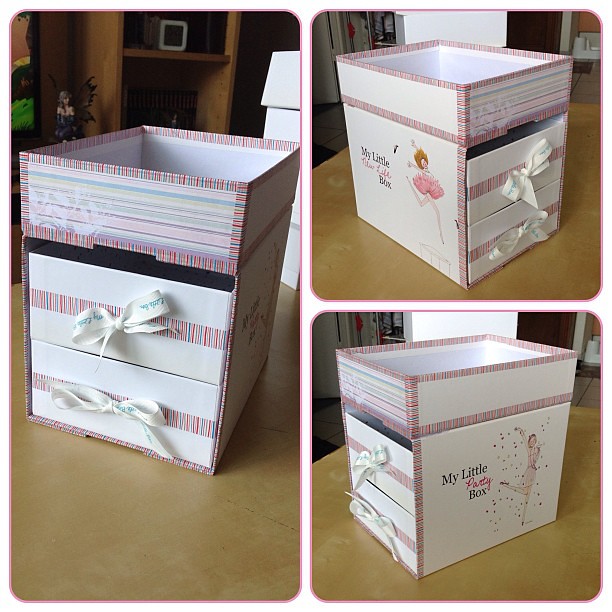The image is a square collage featuring three photos of the same decorative box, arranged with one elongated photo on the left and two equally sized photos stacked vertically on the right. All images have curved corners and light pink borders. The left photo showcases the white box with rainbow-colored borders, pink and green stripes, and two drawers with white bows, sitting on a smooth, light brown floor. It appears slightly tilted forward to the left, against a backdrop that includes a wooden cabinet and other items. The top right photo highlights the side of the box that reads, "My Little Box," adorned with a ballerina figure dressed in a pink tutu with reddish-brown hair and her feet aloft. The bottom right photo depicts the side labeled "My Little Party Box," featuring a woman in a pink dress throwing confetti with one leg raised. Surrounding the box are additional decorative elements like a large fairy, a lamp, and a bookshelf, enriching the scene.